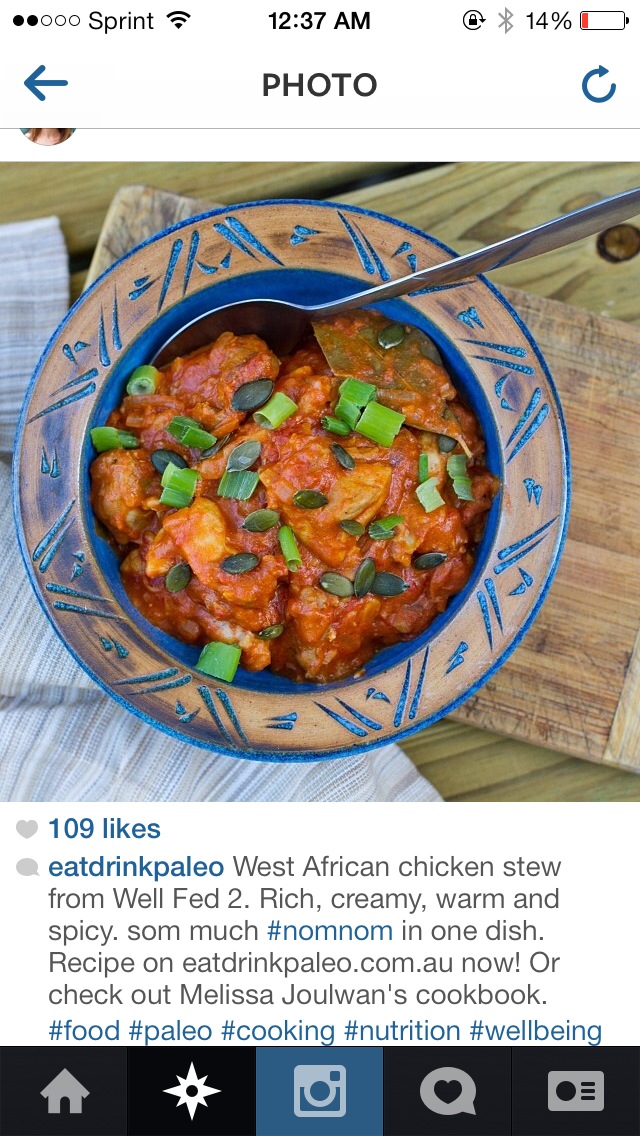The image is a snapshot of a social media post taken from a cell phone screen, displaying a post from Instagram. The overlay text at the very top of the screen reads "Sprint 12:37 a.m." with a battery level at 14%. Below this, the label "PHOTO" appears in all caps. The focus is a large, detailed, top-down photograph of a vibrant West African chicken stew. The stew sits in a visually striking bowl that is beige with blue designs and rests on a rustic, wooden table with a white striped napkin partially visible on the bottom left. The stew appears rich and thick with an inviting orangey-red hue, dotted with green spring onions and what looks like black seeds sprinkled on top. A spoon is tucked into the dish, ready for serving. 

Below the image are the social media post details: it states that the post has received "109 likes" and is authored by Eat Drink Paleo. The text enthusiastically describes the stew as "Rich, creamy, warm and spicy," and encourages users to find the recipe on eatdrinkpaleo.com.au or check out Melissa Joulwan's cookbook, "Well Fed 2." At the very bottom of the screenshot, a black horizontal band shows navigation icons including a home, a star, a camera, a heart, and a message bubble, typical of an Instagram interface.